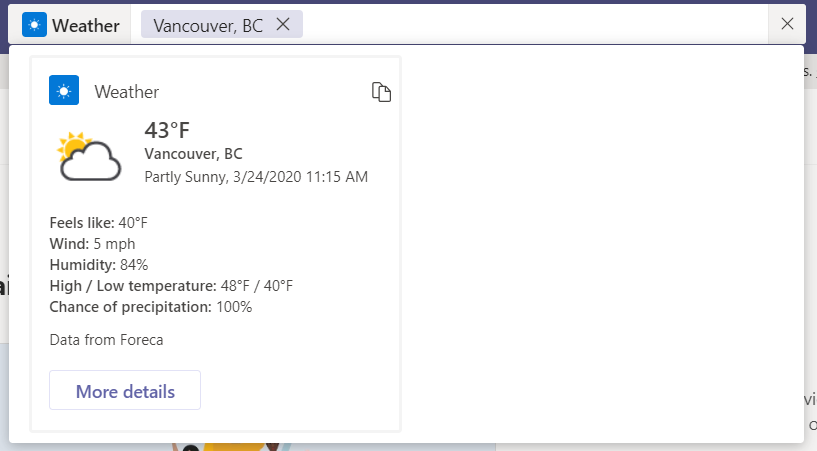The image, a screenshot taken from a computer, features a weather application open on the screen. In the upper left corner, there's a white sun icon within a blue square. Adjacent to this icon, the word "Weather" is written in black print. The user has typed in "Vancouver, B.C.," and there is an "X" next to it that allows the user to clear the input. At the end of the row, another "X" option is available, likely to close the weather search.

The right side of the image is a blank white space, while the left side contains detailed weather information. Below the "Weather" header and the sun icon, it shows the current temperature as 43 degrees Fahrenheit, indicated by an icon of a white cloud with a yellow sun peeking from behind. The text specifies "Vancouver, B.C." and describes the condition as "Partly Sunny." The date and time are displayed as "3/24/2020, 11:15 A.M."

Further details below the cloud icon include:
- "Feels like: 40°F"
- "Wind: 5 MPH"
- "Humidity: 84%"
- "High/Low Temperature"
- "Chance of Precipitation: 100%"

At the bottom of the weather details, there's a button labeled "More Details" for additional information.